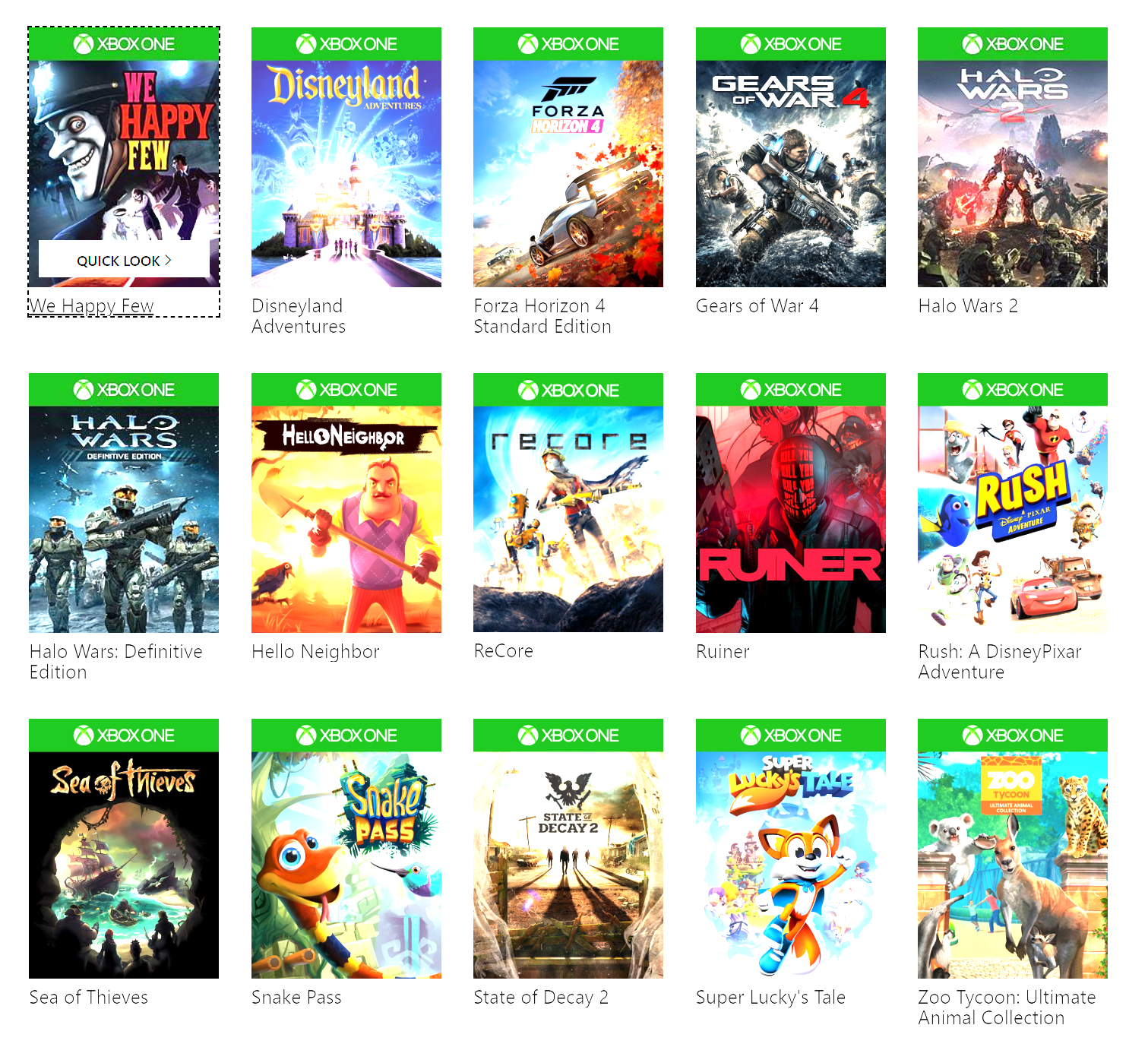The image displays a neatly organized grid featuring 15 Xbox One game titles, arranged in three rows and five columns. Each game's box art is prominently shown. The selection includes a variety of genres and styles, providing a well-rounded representation of the platform's offerings.

Highlighted games include:

- **We Happy Few**
- **Disneyland Adventures**
- **Forza Horizon 4 Standard Edition**: The cover art features a car speeding through a picturesque autumn landscape.
- **Gears of War 4**: Showcases a character armed with a large gun.
- **Halo Wars 2**: Depicts a formidable figure wielding a massive hammer, with soldiers arrayed in the backdrop.
- **Halo Wars: Definitive Edition**
- **Hello Neighbor**
- **ReCore**
- **Ruiner**
- **Rush: A Disney Pixar Adventure**
- **Sea of Thieves**: Its cover art captures a pirate emblem intricately designed with a scene of a sea and pirate ship within.
- **Snake Pass**: Features a strikingly colored snake in orange, black, and white hues.
- **State of Decay 2**
- **Super Lucky's Tale**
- **Zoo Tycoon: Ultimate Animal Collection**

Each box art is creatively designed, making the selection visually appealing. Standouts include Sea of Thieves’ pirate-themed emblematic design and Forza Horizon 4’s autumnal racing scene, exemplifying the detailed and captivating artwork characteristic of these titles.